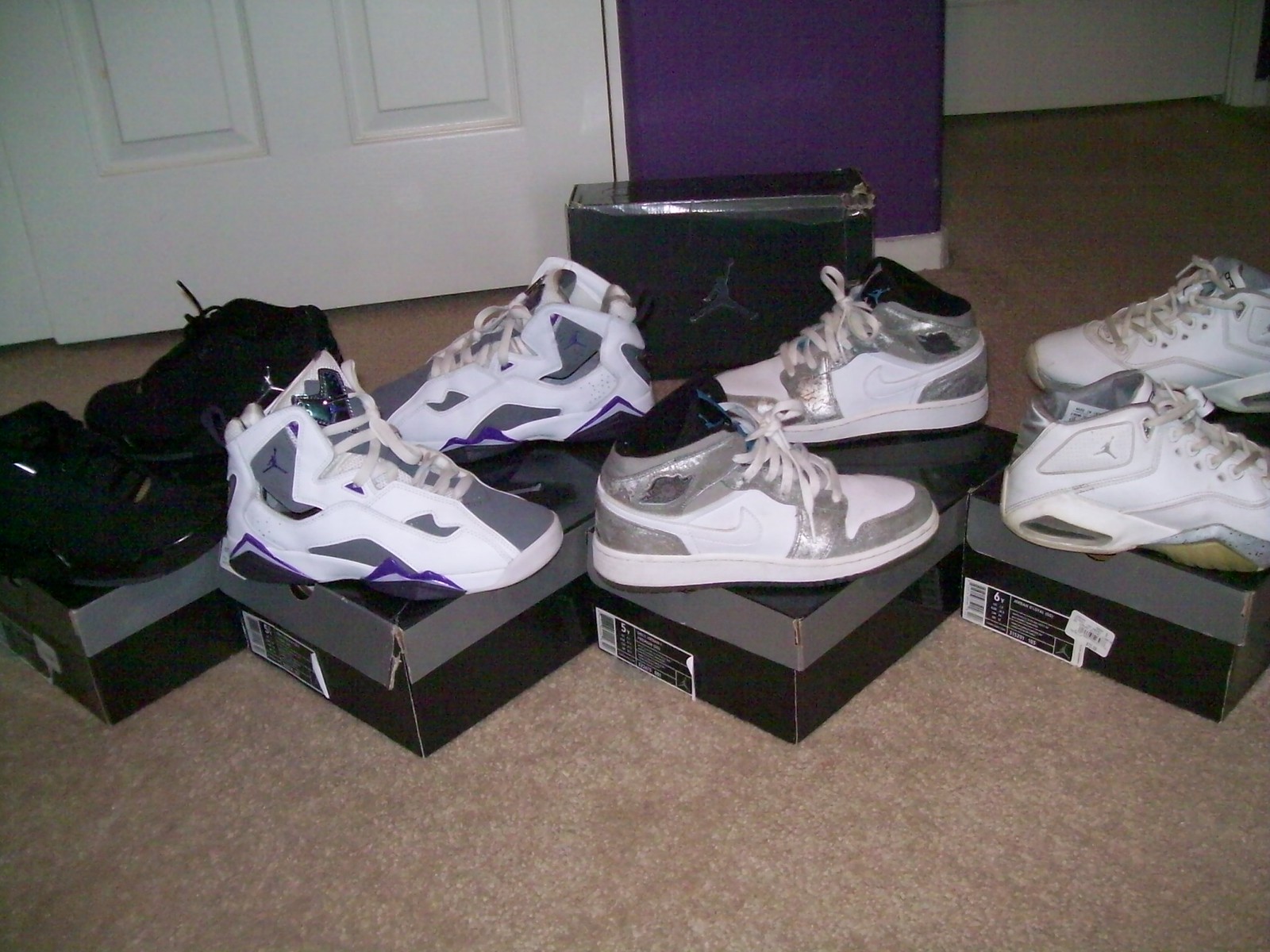This image showcases four pairs of basketball shoes, meticulously arranged atop black and gray shoe boxes positioned on a brown carpet. The boxes are laid out diagonally, their orientation directed to the left and toward the viewer, placed side by side in a coordinated manner. Each pair of shoes is displayed with one shoe facing right in the front and the other facing left in the back. 

From left to right:

1. The leftmost pair features sleek black high-tops, shrouded in darkness which makes it difficult to ascertain their brand, but they exude a classic athletic aesthetic.
2. Next, a pair of Air Jordans strikes a modern, almost futuristic note with a distinctive gray, blue, and white color palette. The signature Michael Jordan symbol adorns the ankle, highlighting their iconic status.
3. The third pair from the left or second from the right showcases a blend of silver and white high-tops with prominent white Nike symbols. These sneakers are crafted with a contemporary edge that appeals to sneaker enthusiasts.
4. On the far right, white Air Jordans command attention with their crisp, clean design accented by subtle yellow tints at the bottom and a gray interior, exuding an aura of elegance and sporty chic.

Each pair is a testament to the fusion of style and functionality that defines today's basketball footwear.